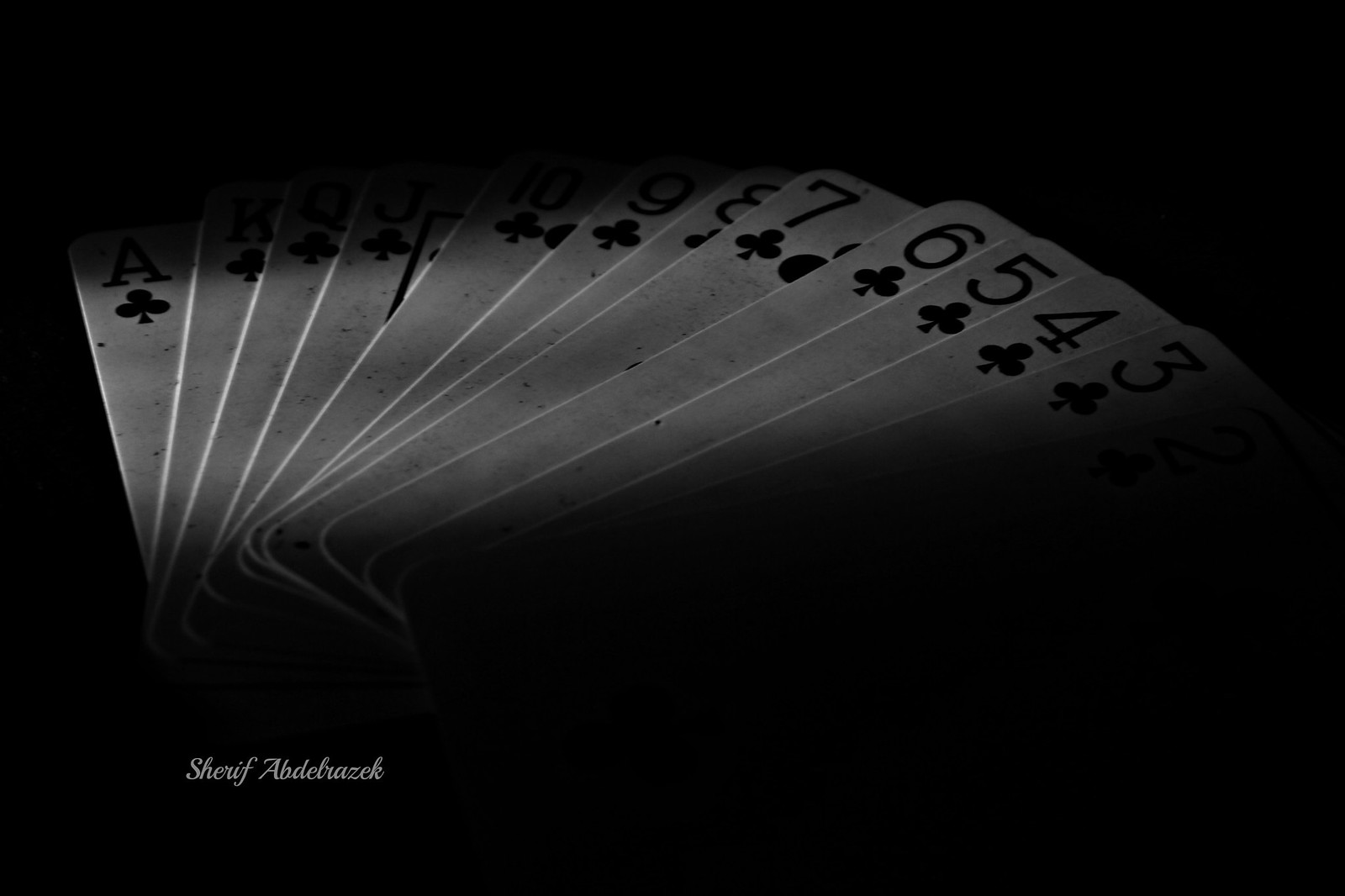A dimly lit photograph showcases a spread of playing cards, all from the suit of clubs, arranged face-up. The visible cards range sequentially from the ace down to the three, although the two of clubs is obscured by shadows. The lighting, subtle and likely filtering through a small or shaded window, illuminates the majority of the cards but leaves the tops and bottoms in darkness. The side-lit scene creates a stark contrast, drawing attention to the crisp details of the visible cards. In the bottom left corner, the phrase "Sheriff Abdelrazak" is printed in small, white font. The play of light and shadow lends a dramatic atmosphere to the seemingly casual spread of shuffled cards.